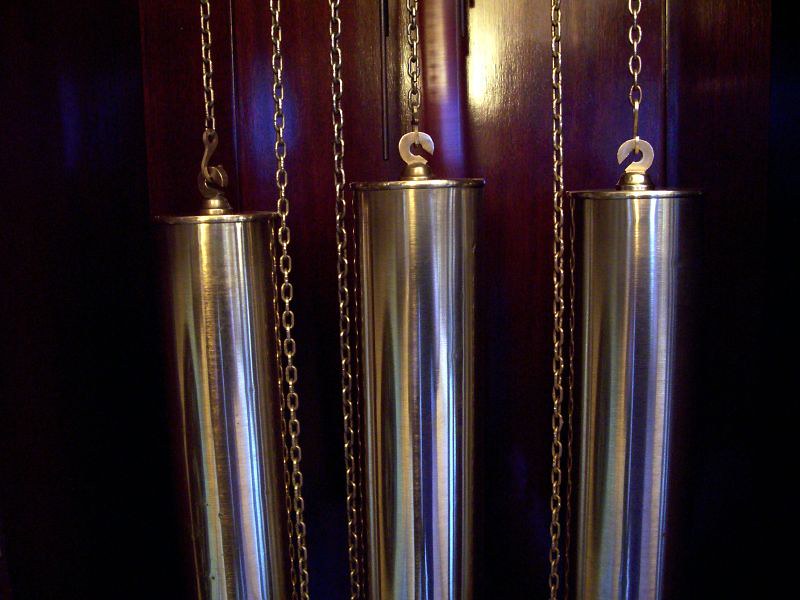In this image, set against a dark background, we see three large silver cylindrical weights that are likely components of a clock mechanism, such as grandfather clock weights or a balancing device. The background transitions from black on the outer edges to dark brown, hinting at a finely finished wooden panel or the interior of a piece of furniture like a drawer or wardrobe. Each weight is suspended by a lightweight, silver chain with rounded loops at the top for attachment. The chains extend both upwards out of frame and between the cylinders, suggesting there might be additional weights or mechanisms beyond the visible portion. The central focus is on these shiny metal weights and their intricate yet minimalistic chain assembly, set against the contrasting dark mahogany wood, which imbues the scene with a vintage, mechanical aesthetic.